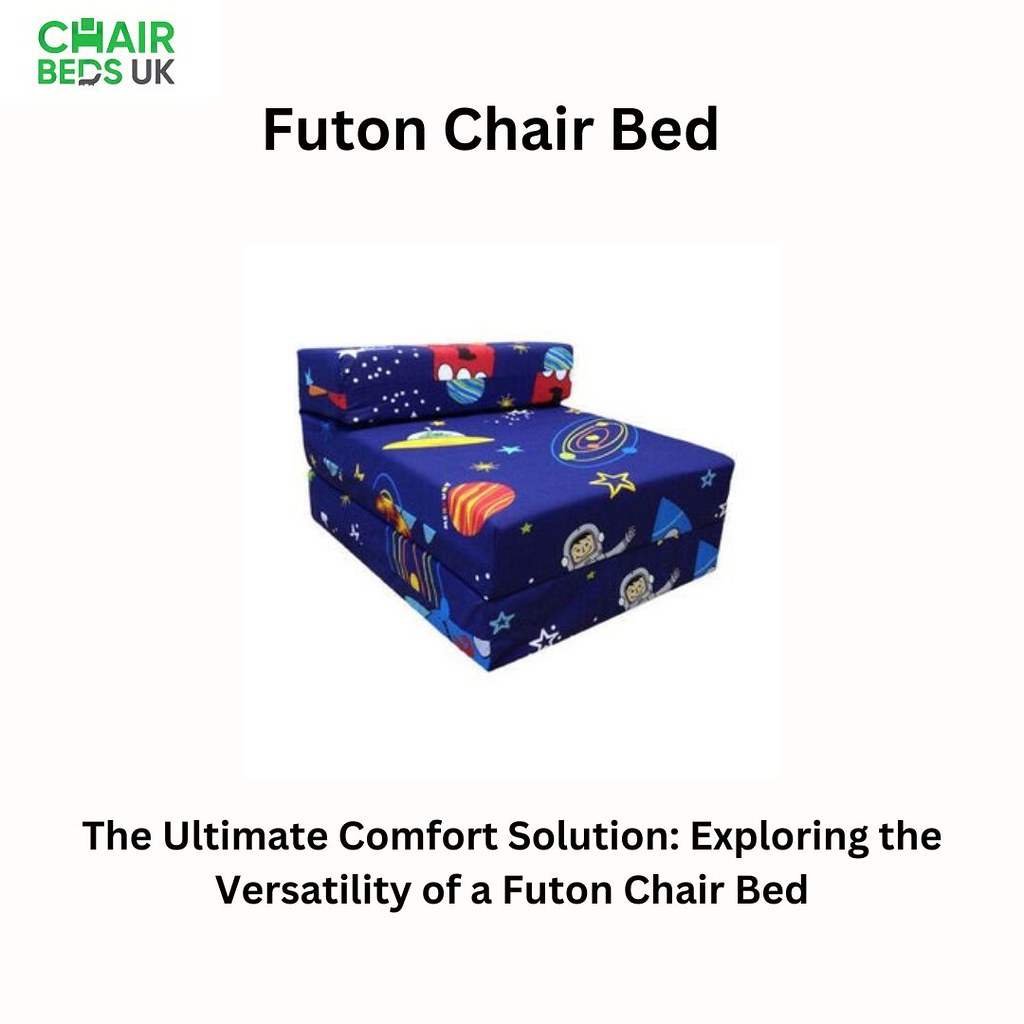This image features a futon chair bed prominently displayed against a white background. At the top left corner, text reading "ChairBedsUK" appears, where "Chair and Beds" is in green text, and "UK" is in gray. Notably, the letter "H" in "Chair" is styled to resemble a sofa, while the bottom of the "D" in "Beds" looks like a leaning chair. In the center top, bold black text states, "Futon Chair Bed."

The image showcases a partially extended futon chair bed angled slightly to the right. Surrounding the bed are whimsical space-themed illustrations, including an astronaut, a flying saucer, Jupiter, various stars, and a solar system motif featuring red and yellow planets and constellations.

Below the image of the bed, a caption reads: "The ultimate comfort solution, exploring the versatility of a futon chair bed." The futon bed's noticeable thickness and shorter length hint at its dual functionality as both a chair and a bed.